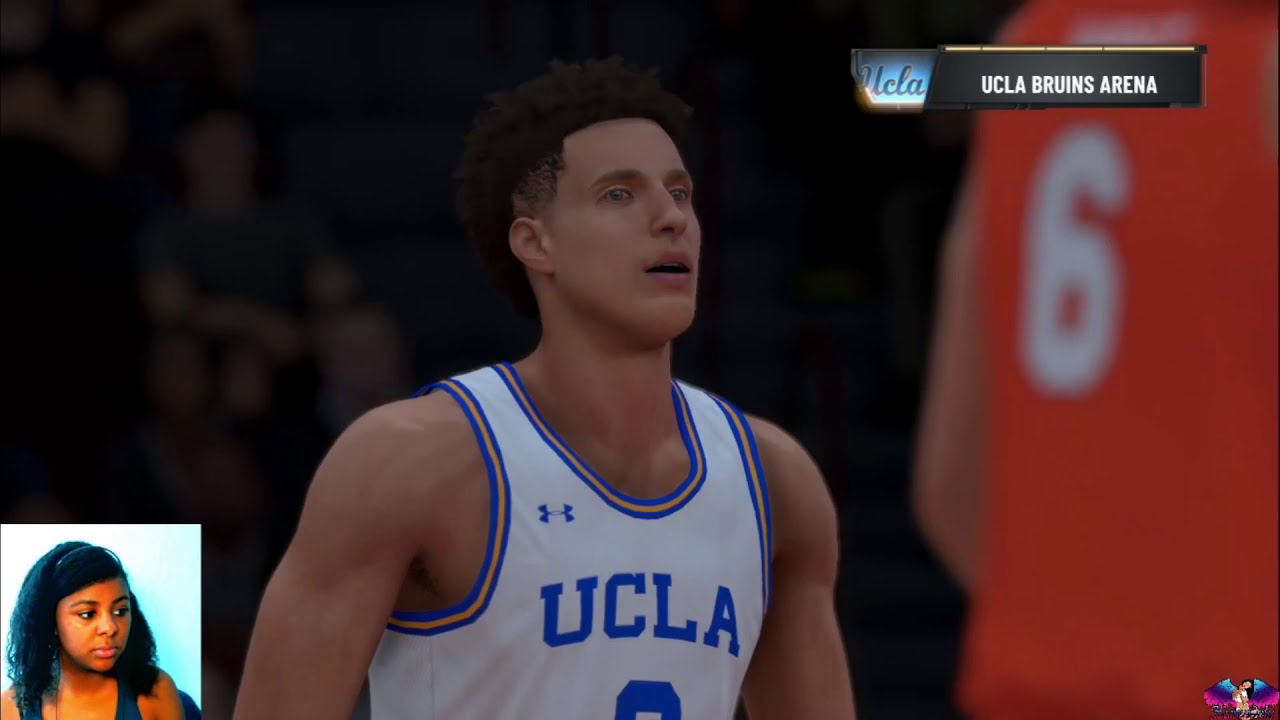The image is a horizontal rectangular screenshot from a basketball video game stream. In the lower left-hand corner, there's a small inset of the streamer, a young black woman with long, curly black hair, wearing a black tank top and black headphones. She appears focused, possibly looking at her monitor. The streamer’s dark complexion contrasts with the vivid colors of the game behind her.

The main focus of the image is a detailed close-up of a UCLA basketball player at the center. The player, a young man with short, slightly curly brown hair, and bright eyes, is captured looking off towards the right with his mouth slightly open. He has muscular arms and is donning a white team jersey with blue and gold stripes, featuring an Under Armour logo on the upper right chest and "UCLA" in large blue letters across the chest. Though partially visible, his jersey number appears to be eight.

To the right of the central player, there is a blurry view of another player wearing an orange jersey with the number six visible. The background reveals a packed arena with spectators on the bleachers, including the faint outline of a man holding a child. In the upper right corner of the screen, white text reads "UCLA Bruins Arena" against a black background.